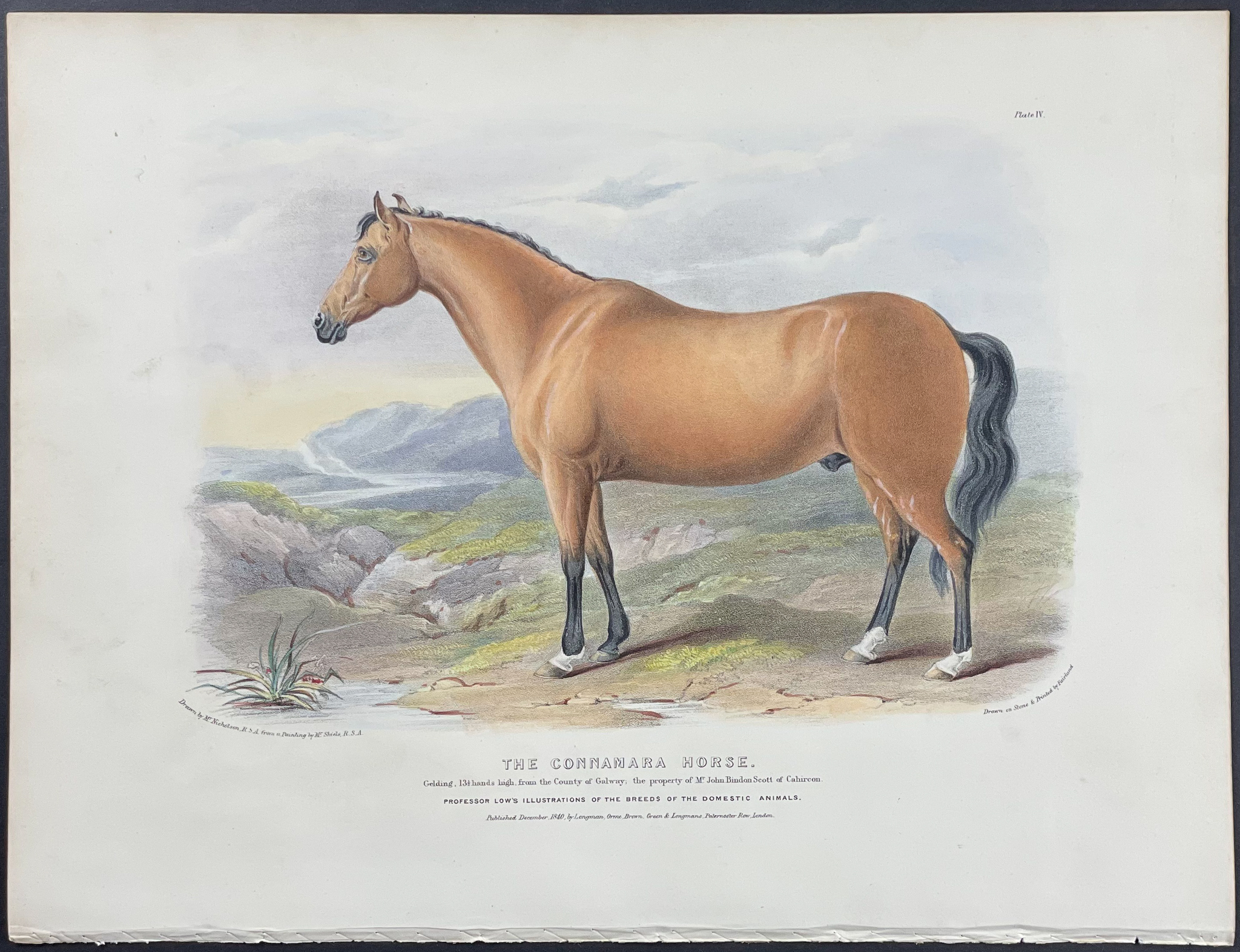The image is a detailed painting framed in black, resembling a page from a book. At its center, a light brown horse with black legs, a black mane, and a black tail stands in profile, facing and looking slightly to the left. The horse features white socks on three of its legs. Its ears are perked up, and it appears attentive. The background is a muted, pale landscape with mountains, water, and a gray sky, along with some rocks and patches of grass. To the left, there's a small patch of water and a plant or seaweed. Below the painting, in capital letters, it reads "THE CONNEMARA HORSE," with three small, unreadable lines of text beneath it. The overall scene is enriched with colors such as white, gray, silver, green, yellow, red, orange, brown, and black, creating a vivid, multi-colored artistic piece.